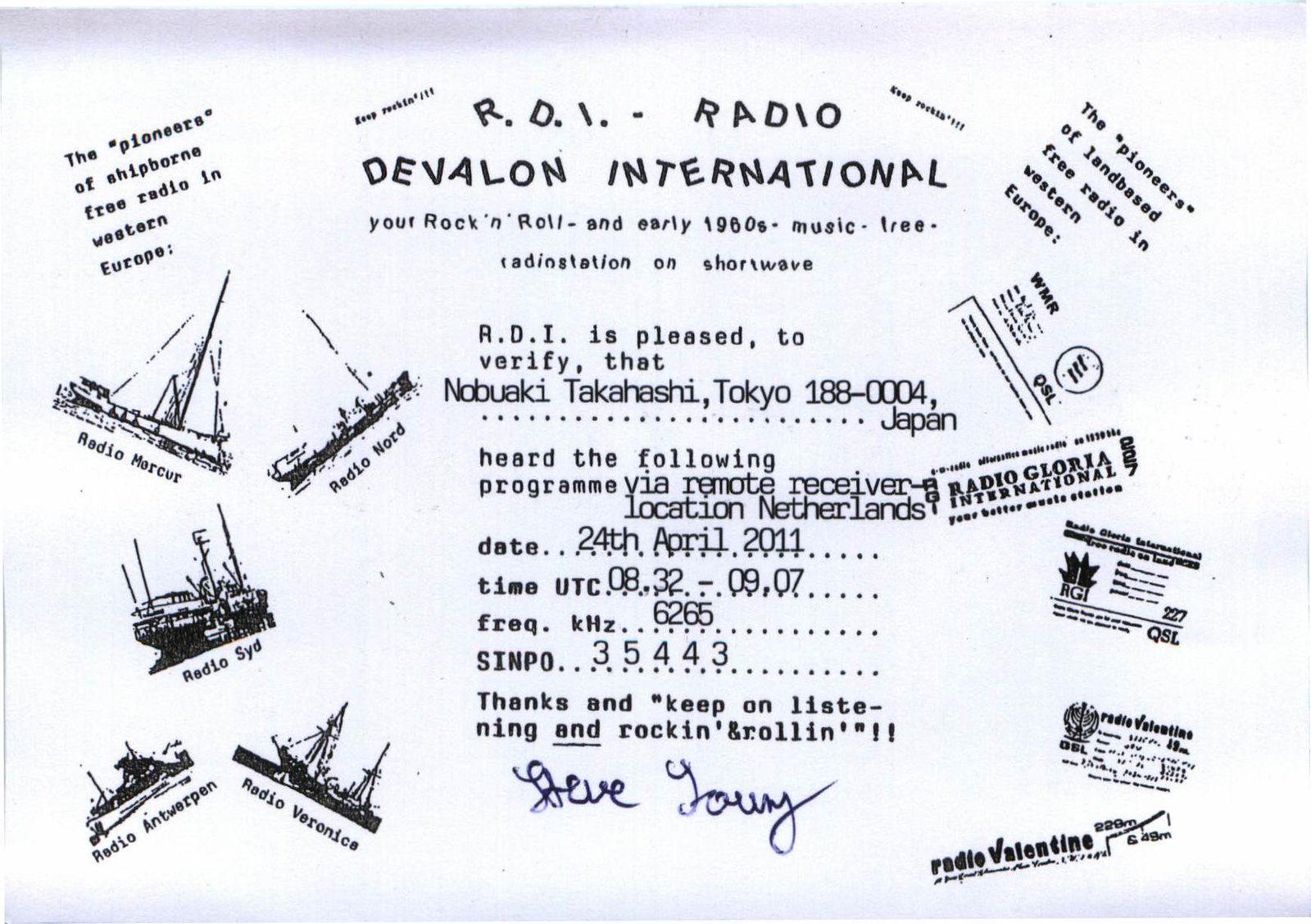The promotional flyer for "RDI Radio Devilon International" is a busy and vibrant advertisement for a shortwave radio station specializing in rock and roll and early 1980s music. The entire flyer measures approximately four inches tall by six inches wide, featuring a light blue background that darkens slightly at the top and bottom. The top of the flyer boldly states: "RDI Radio, Devilon International: Your rock and roll and early 1980s music free radio station on shortwave." The flyer is cluttered with various images and text, contributing to its lively appearance. On the left side, five ship illustrations resembling stamps are arranged at different angles, each accompanied by names such as Radio Mercut, Radio Nord, Radio SID, Radio Antwerpen, and Radio Veronica, with a caption reading "The pioneers of ship-borne free radio in Western Europe." The right side features logos and stamps of other radio entities like WNR QSL Radio Gloria International and RGI QSL Radio Valentin, under a heading that says "The pioneers of land-based free radio in Western Europe." In the center, it verifies the reception of a broadcast by Nobuaki Takahashi in Tokyo, dated April 24th, 2011, via a remote receiver in the Netherlands. The Signal-to-Noise Ratio (SINPO) is listed as 35443, and a message encourages continued listening with a signature from Steve Young in blue cursive.